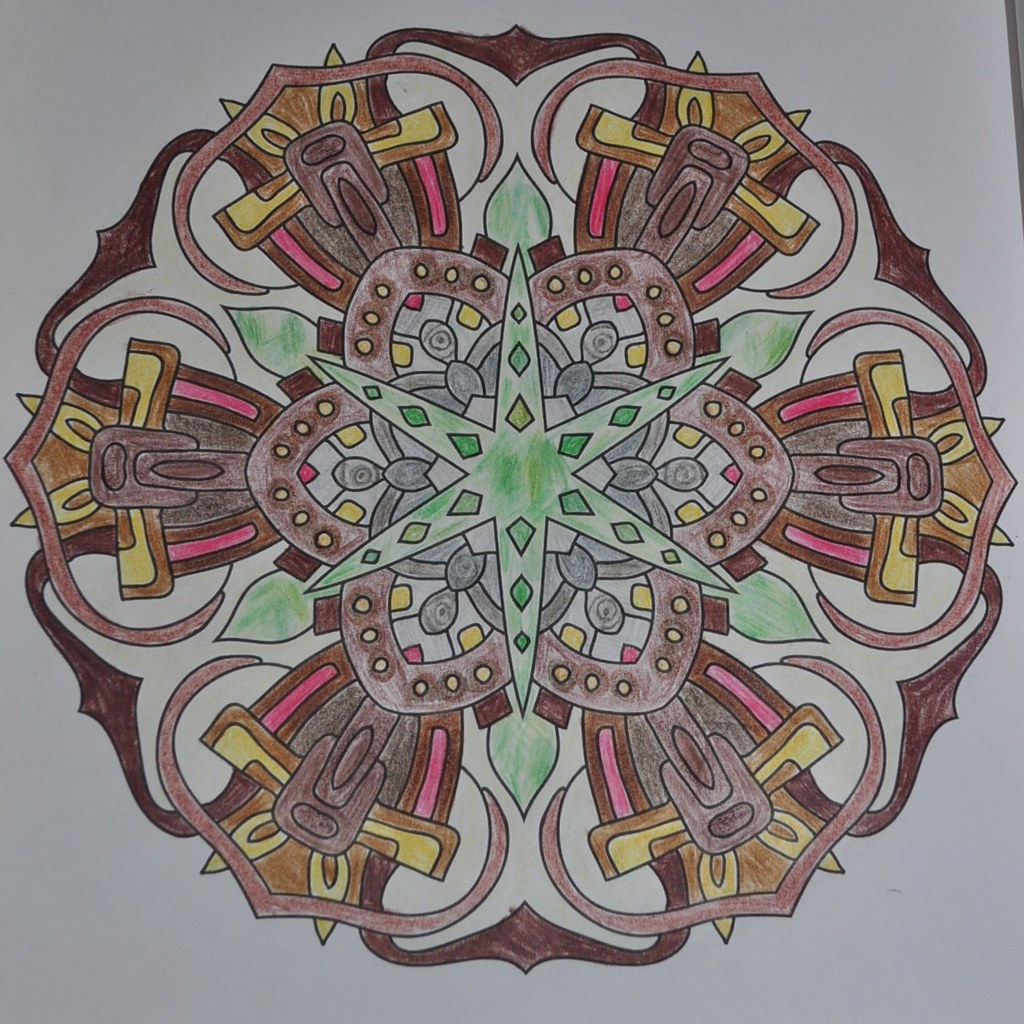This vibrant painting, set against a light gray background, depicts a detailed and colorful medallion. Central to the medallion is a green, six-pointed star, whose points are adorned with delicate green leaves. Intricately arranged mosaic tiles embellish the top of the star, adding texture and depth. Surrounding this core are various colorful and shapely figures, extending outwards to form the next layer of this elaborate design. Along the outer edge, the medallion features six shield-like shapes in shades of brown and pink, seamlessly integrated into the composition. The entire medallion is bordered by a dark brown rim, framing the intricate artwork within. The harmonious blend of colors and shapes showcases the artist's meticulous attention to detail and creative vision.